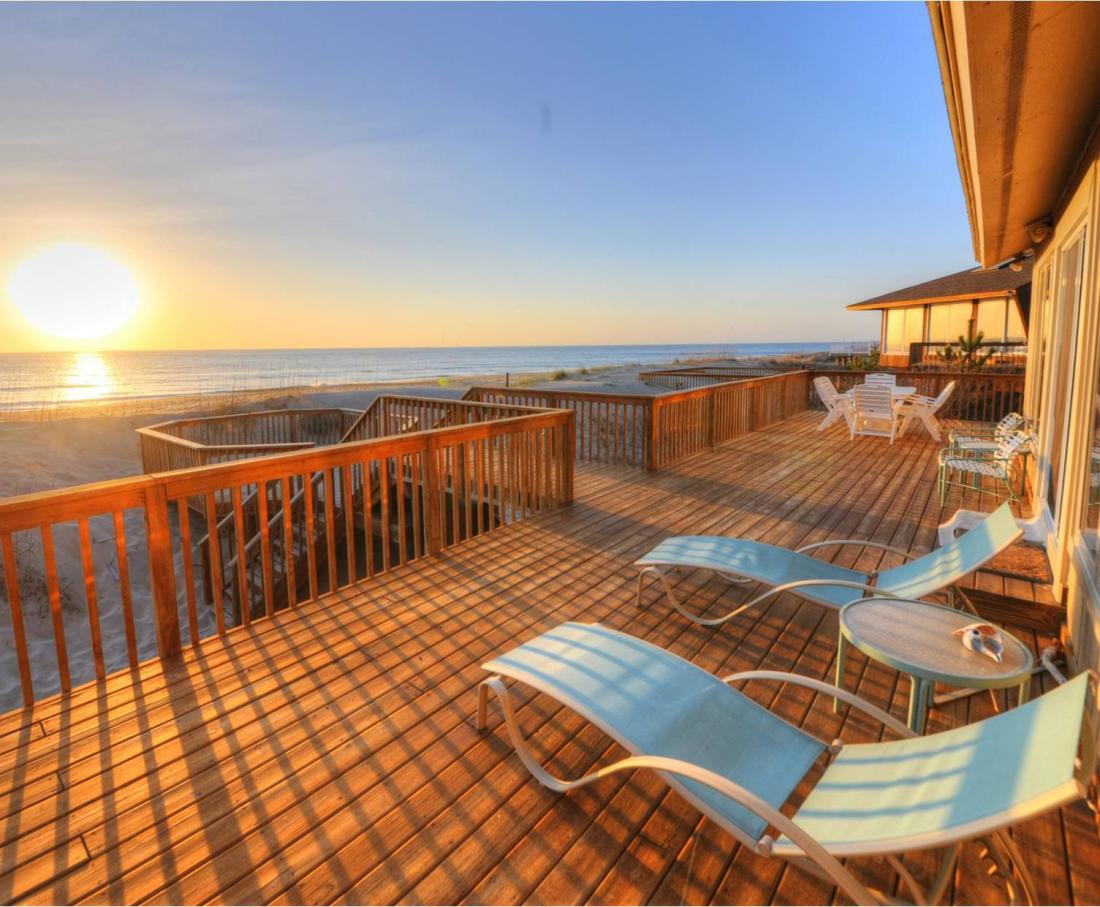This photograph captures a stunning beachfront property at sunset. The primary focus is a large, brown wooden deck attached to the house, with natural wood finishes that show no signs of gloss or added treatments. The deck, approximately seven feet off the ground, offers multiple lounging options, including two wavy blue reclining chairs, a small circular table with what appears to be either a wooden or glass top, and a distant cluster of wooden and white chairs surrounding a table. Toward the right, glass sliding doors lead into the house, which features a secondary, lower octagonal deck connected by a short pathway. This lower deck sits close to a set of stairs that lead directly to the sandy beach. The surrounding scenery includes another property visible across from the house. The photograph boasts a captivating ocean view with the sun setting toward the left, casting a warm yellow glow over the scene, though the sky remains a dim blue with sparse cloud cover. The sunlight reflects on the water, creating a smaller shadowy orb directly beneath the sun itself. This serene and picturesque setting is framed by the gentle waves and the inviting beach, making it a perfect seaside retreat.